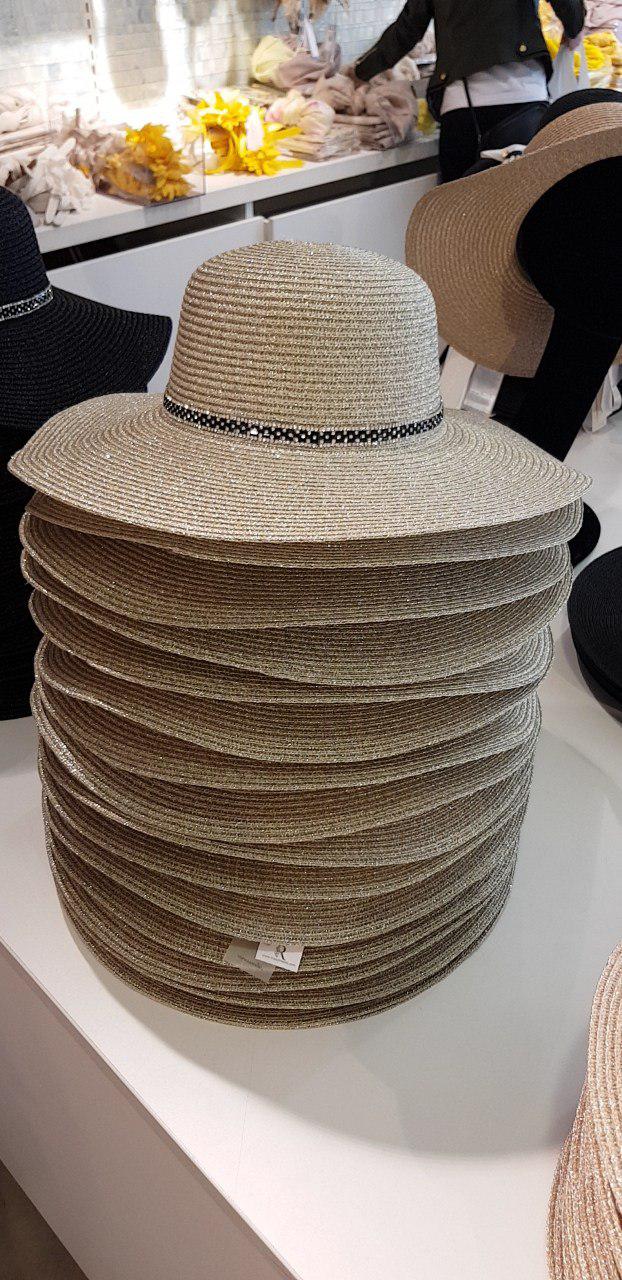This color photograph, taken in portrait mode, captures a detailed view inside a boutique. In the foreground, there is a white rectangular base display stacked with at least 16 tan straw hats, each featuring a black sequin band around the base. Adjacent to this stack, a black straw hat and another hat positioned on a black mannequin head and neck form mirror the style. In the background, a shopper dressed in a black jacket over a white T-shirt and black pants peruses through what appear to be scarves, organized in sections along the store wall. The display sits on a white contemporary countertop with matching cabinetry below, and price tags are visible on each of the hats, though their prices are not discernable. A secondary display in the distance contains bins with yellow and white headbands. The overall scene vividly captures the shop's meticulous organization and diverse yet cohesive hat collection.